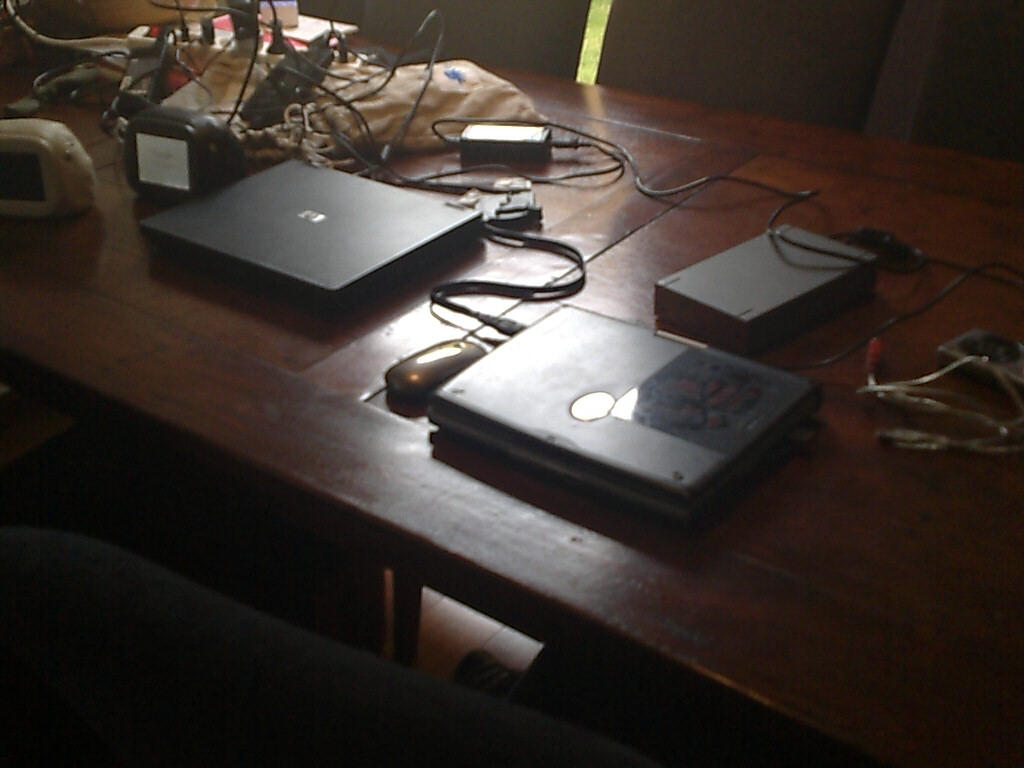The photograph captures a dimly lit scene of a large wooden desk, possibly made of dark mahogany. On the desk, there are two black laptops prominently displayed amid a disorganized array of electrical devices and peripherals. The older model laptops appear thicker, with one possibly featuring a CD or optical drive. Tangled wires cascade from a power strip, mingling with adapters and chargers, creating a chaotic mess. In the upper section of the photo, a white bag sits on the table, near what looks like semi-open window shutters revealing a glimpse of greenery, possibly a lawn. The image is slightly blurred and shadowy, with additional items including what may be the backs of three chairs visible at the top and another chair barely visible on the side. The photo extends into darkness at the bottom, obscuring further detail.